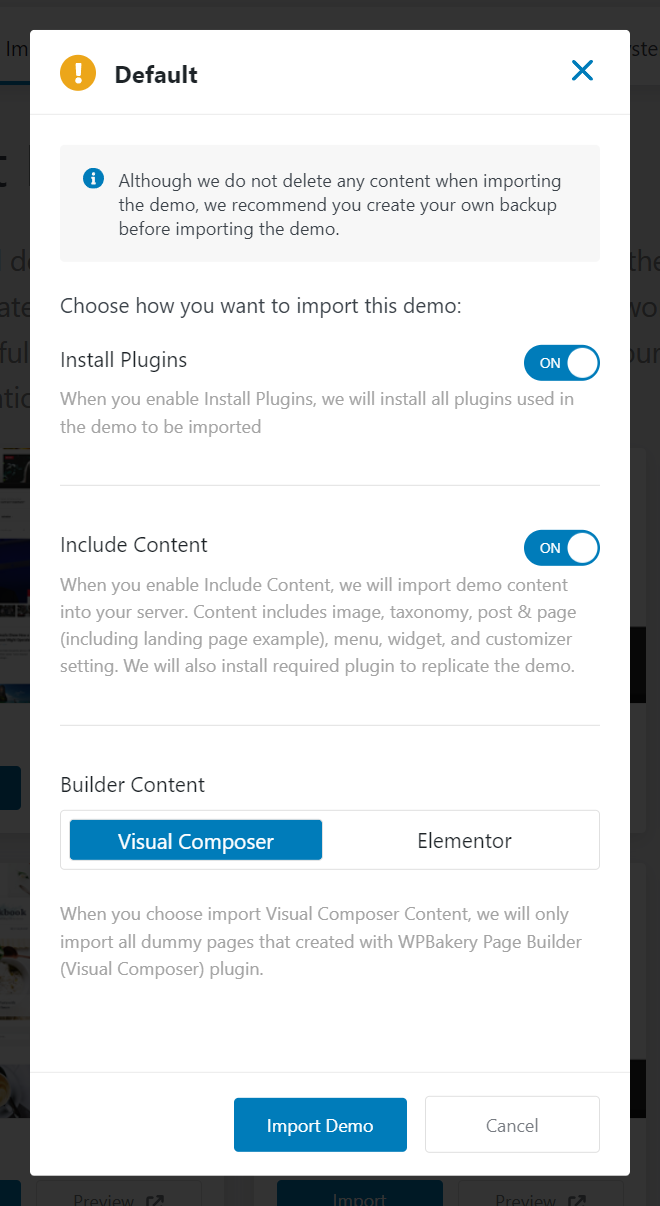**Detailed Screenshot Description:**

This screenshot displays a user interface for importing a demo on a website. Here's the detailed breakdown of the image from top to bottom:

1. **Header Section:**
   - In the top-left corner, there is an exclamation point within a golden circle. To the right of this icon, the word "default" is displayed in black text.

2. **Notice Box:**
   - Below the header, a text box contains a cautionary message: "Although we do not delete any content when importing the demo, we recommend you create your own backup before importing the demo."

3. **Import Options:**
   - The next section prompts the user to "Choose how you want to import this demo." 
   - **Install Plugins Option:**
     - There is a toggle button labeled "Install Plugins," which is turned on. 
     - The associated text reads: "When you enable Install Plugins, we will install all plugins used in the demo to be imported."

   - **Include Content Option:**
     - Below, there's another toggle button labeled "Include Content," which is also turned on.
     - The explanatory text under this option states: "When you enable Include Content, we will import demo content into your server. Content includes images, taxonomy, posts and pages, menu, widgets, and customizer settings. We will also install required plugins to replicate the demo."

4. **Content Builder Selection:**
   - This section is titled "Build the Content."
   - Two builder options are presented: **Visual Composer** and **Elementor**. 
   - "Visual Composer" is highlighted in blue, indicating it is the selected option.
   - The text beneath both options explains: "When you choose Import Visual Composer content, we will only import our dummy pages that are created with WP Bakery Page Builder plugin."

5. **Action Buttons:**
   - At the bottom of the screen, there are two buttons. 
   - The "Import Demo" button is blue, suggesting it is the primary action. 
   - The "Cancel" button is white.

This detailed description covers all text and elements present in the screenshot, providing a clear understanding of the interface and its functionalities.